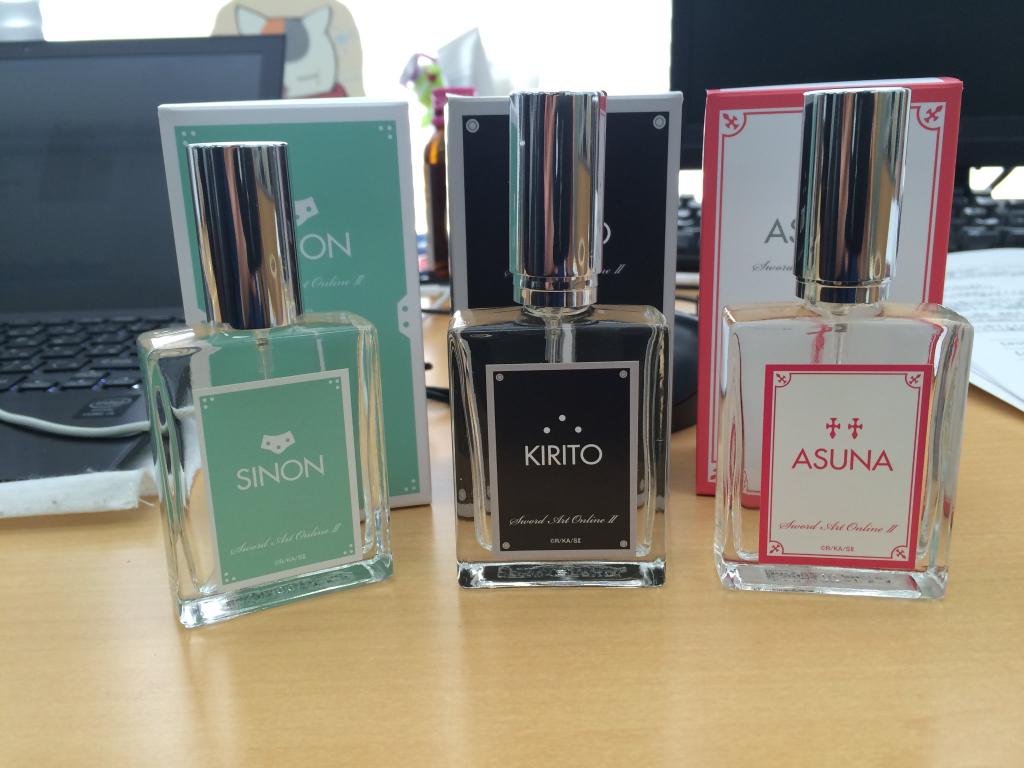This photo features three clear glass perfume bottles arranged on a light brown table. Each bottle has a silver cylindrical cap and a rectangular body, clearly displaying its label which matches the color of its packaging behind it. The bottle on the left has a green label with the word "Xenon" and a cat face above it. The middle bottle features a black label with "Kirito" and a triangle of three dots. The rightmost bottle showcases a white label with pink edges, adorned with the name "Asuna" and two shore symbols. Each bottle's respective packaging is directly behind it. In the background, there are two computer screens: to the left, an open Windows laptop with a gray cord across its blank screen, and to the right, a standalone computer monitor. The bottles and their aligned boxes provide a striking contrast against the light brown table, while the tech setup in the background adds a modern touch to the scene.